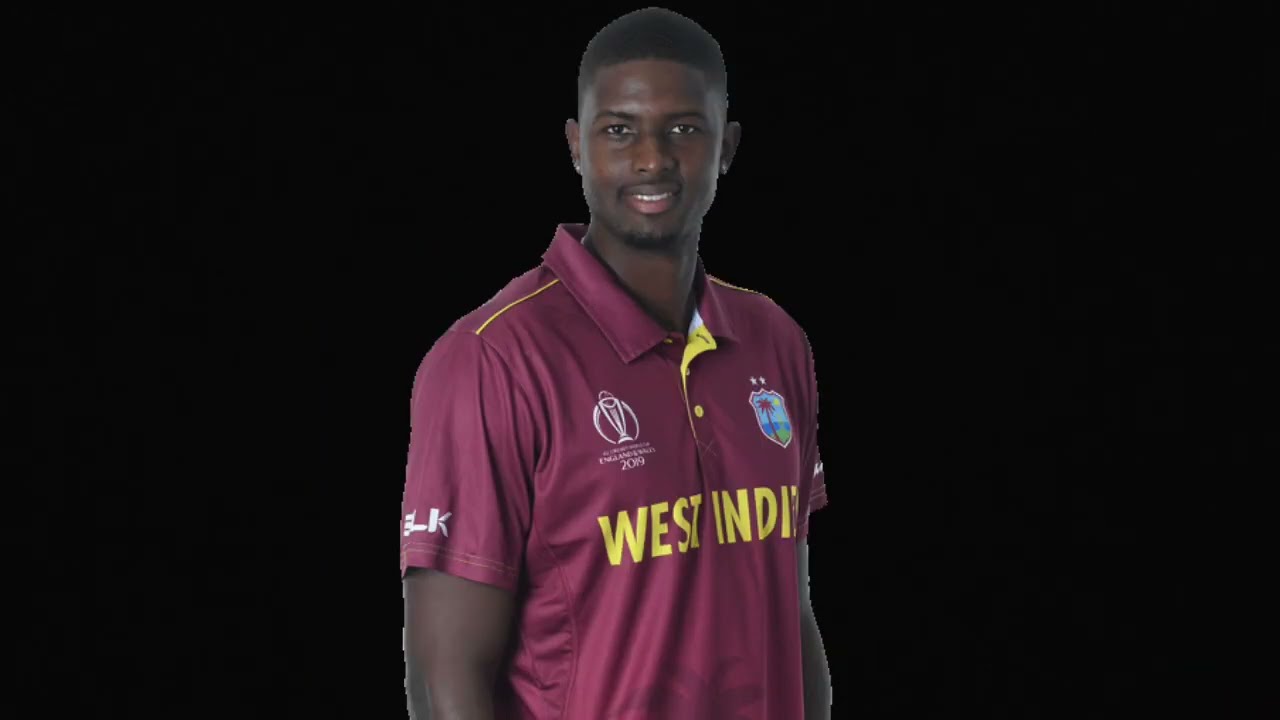In this posed landscape photograph against a black background, a man stands centered and cut off at the waist. The man, who appears to be in his 20s, is an African-American with dark black skin, short black hair, a mustache, and a goatee. He stands slightly angled to the right, but his head is turned to face forward, looking directly into the camera with an open-mouthed smile that reveals his pink lips and a glimpse of his upper row of white teeth. He is wearing a maroon collared shirt with short sleeves that reach halfway down his biceps. The shirt features yellow text that reads "West Indies" across the chest and has yellow lines on the front of each shoulder. There are two emblems on the shirt: the left emblem is white, and the right emblem resembles a badge depicting a beach scene with a palm tree and a yellow background. Above his right bicep are the letters "BLK" written in white. There are no visible earrings, piercings, or tattoos on him. The photograph's clean, dark background and the precise placement of the man suggest a professionally posed portrait.